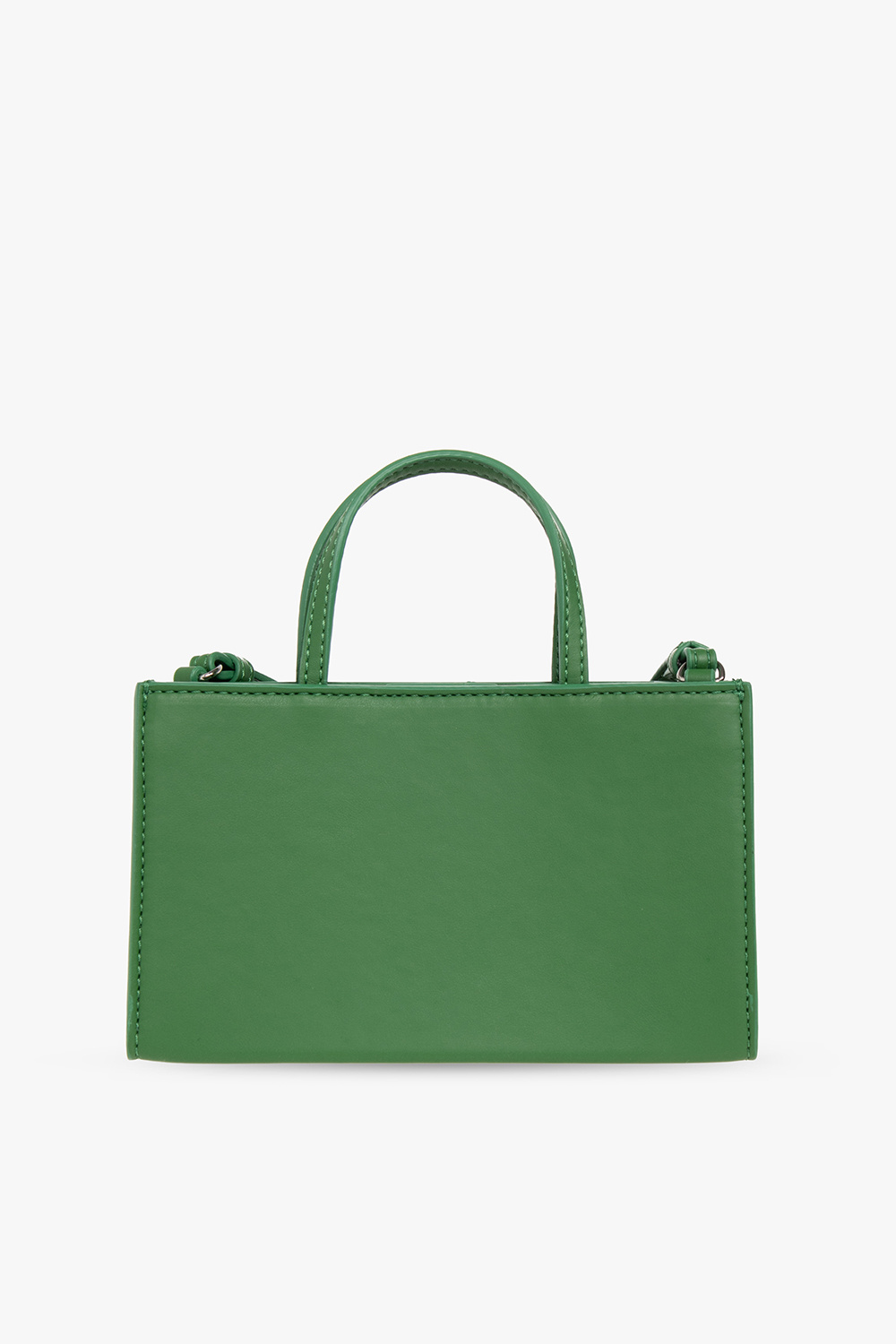This photograph showcases a kelly green purse set against an all-white backdrop. The purse is rectangular in shape and features simple, prominent stitching around the outer edges. It is equipped with two short, arched handles, each reinforced by two lines of stitching to ensure durability. Additionally, the purse includes two longer straps designed to convert it into a shoulder or crossbody bag, with silver rings attaching these straps to the purse. Although the longer straps are partially out of view, their presence is unmistakable. The bag, devoid of any intricate designs or textures, appears small and likely suited for carrying a limited number of items, making it an ideal accessory for a fun evening out.